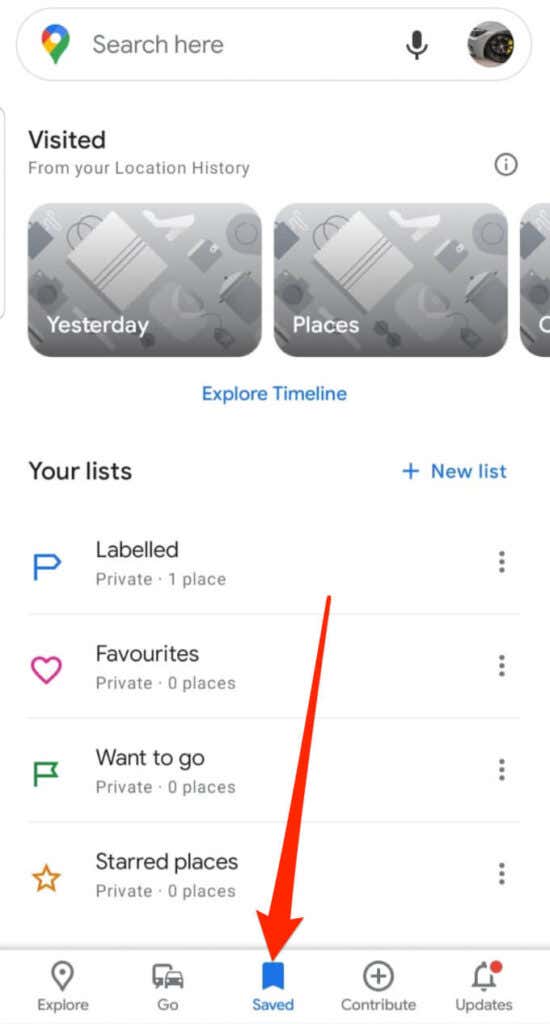The image appears to be a screenshot from an iPhone, displaying the Google search interface. At the top of the screen, the iconic Google logo is visible, featuring its recognizable colors: green, blue, red, and gold. Adjacent to the logo are a microphone icon and a round icon resembling a black circle with several dots inside it.

Beneath the search bar, which is represented as a large white oval with the prompt "Search here," there is a section titled "Visited." This section is outlined by a subtle light gray bar and includes the text "from your location history." A gray box displays "Yesterday," followed by the word "Places," which is partially cut off but includes an accompanying image. This section features black and white icons depicting shopping-related items like a bag and a shoe.

Further down, there is a blue link labeled "Explore timeline." Below this link is the "Your list" section, indicated in gray text, with an "Opposite that" new list option marked by a plus sign. Here, various categories are listed: "Labeled," "Favorites," "Want to go," and "Starred places," each with its respective icon – a blue "P" for Labeled, a heart for Favorites, a green flag for Want to go, and a yellow star for Starred places. 

At the bottom of the screen, five navigation icons labeled "Explore," "Go," "Saved," "Contribute," and "Updates" are visible. The "Updates" icon has a red circle indicator. Finally, a prominent red arrow points downward towards the "Saved" button, suggesting that tapping this button will allow users to explore their timeline shown in the pertinent section above.